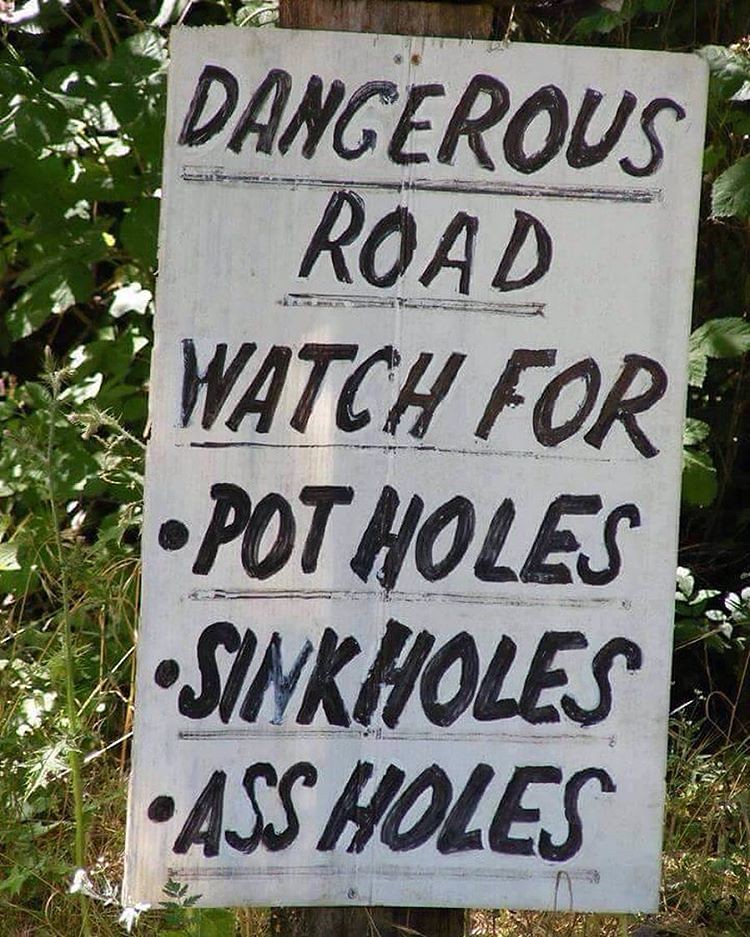The close-up image depicts a homemade, white rectangular sign weathered by time. The sign is affixed to an older utility pole with Phillips head deck screws at the top and bottom, and possibly a nail in the center. It warns: "Dangerous Road. Watch for potholes, sinkholes, assholes." Each warning - "potholes," "sinkholes," and "assholes" - is accompanied by a bullet point and underlined. The text is painted in a black, freehand brush style, giving it a rough, somewhat washed-out appearance. The background is filled with dense, overgrown vegetation, including grass, weeds, and leaves, all illuminated by sunlight streaming from the top left of the image.